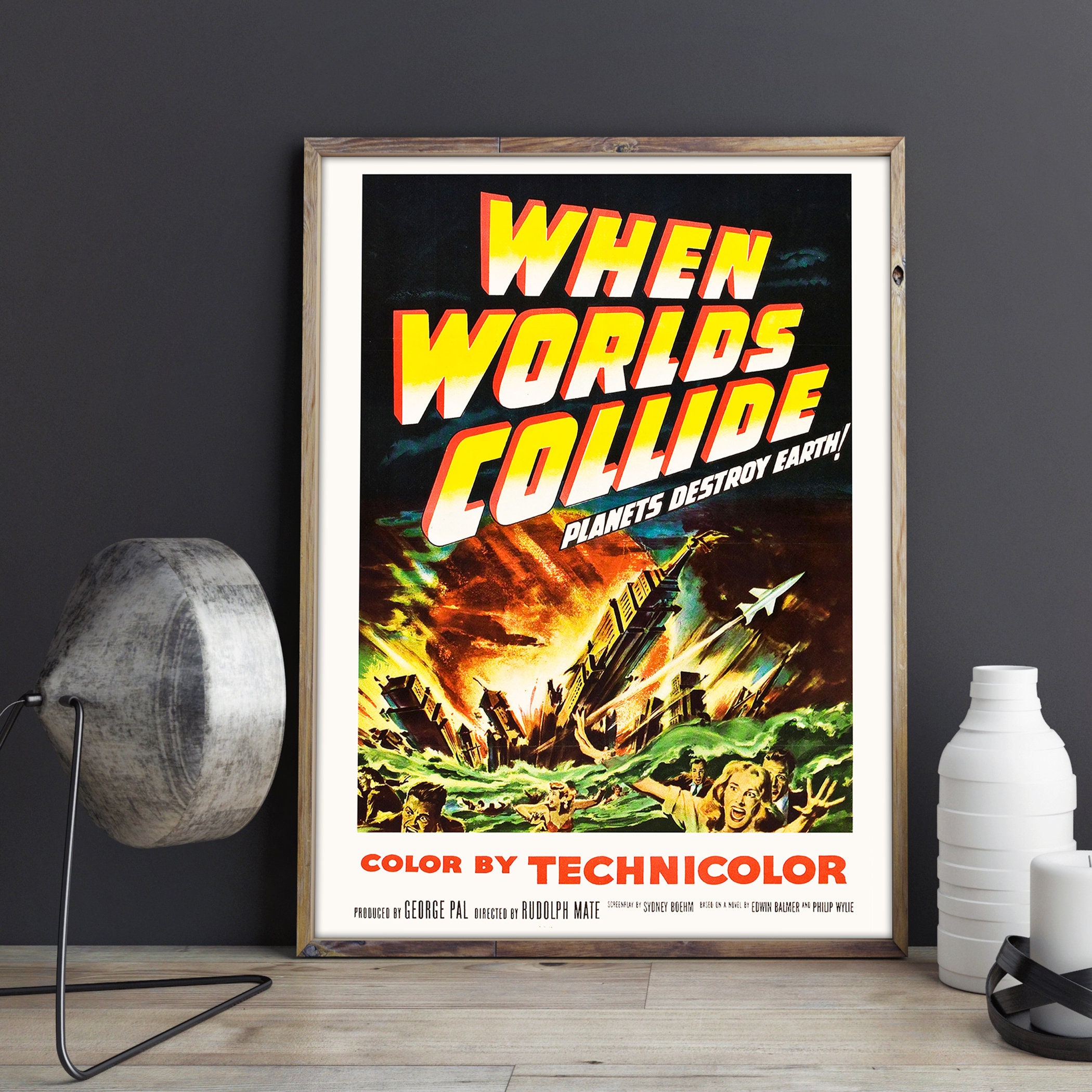The image is a perfectly square photograph of a framed movie poster against a very dark gray wall. The frame itself is gray, encasing a poster that has a predominantly white background. Prominently featured within the poster, large yellow, white, and orange letters declare "When Worlds Collide: Planets Destroy Earth." Below this, the text "Color by Technicolor" appears in orange, followed by additional black text. The central imagery depicts a dramatic scene with people screaming, a planet crashing into a building, airplanes, and water, all set against a black background. At the bottom of the scene, there's a distinct horizontal feature, possibly a gray or grayish tile that might be wood. To the left of the frame is a light fixture, while to the right, there is a white bottle and a white candle, adding subtle elements to the overall composition.